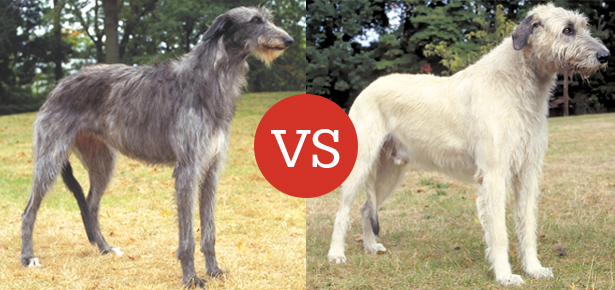The image is a horizontal rectangular composition featuring two adjacent square photos of dogs in a grassy field with a backdrop of dense trees. Both dogs, which appear to be of the same breed with pointed faces, are standing with their right shoulders facing the camera. The dog on the left is gray, while the dog on the right is white with some gray on its ears and body. Both animals have their tails down; the gray dog's tail is behind one of its legs, while the white dog's tail is between its legs, suggesting a less confident or unhappy demeanor. Where the two photos meet, there's a prominent red circle with the letters "VS" in white. The scene suggests a comparison between the two differently colored dogs, possibly asking the viewer which one they prefer.